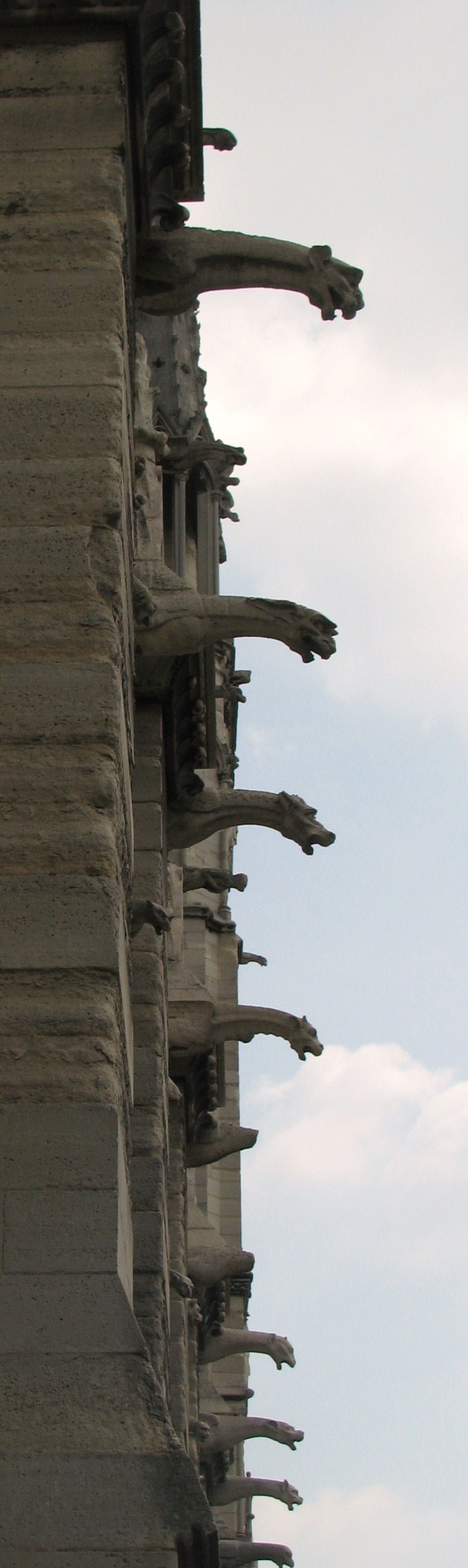The photo captures a tall, narrow building shot from the ground up, likely situated in a historic European locale. The multi-story structure, made of weathered gray stone with some tan hues, features an array of grotesque sculptures jutting from its walls. These sculptures, resembling dragon-like or dog-like creatures with long necks and large ears, have open mouths as if howling towards the pale daytime sky filled with fluffy white clouds. The arrangement includes eight prominent beastly heads aligned in a sequence, creating an eerie and imposing facade. The overall color palette of the image is dominated by the gray and brown tones of the building, contrasting with the light blue sky.